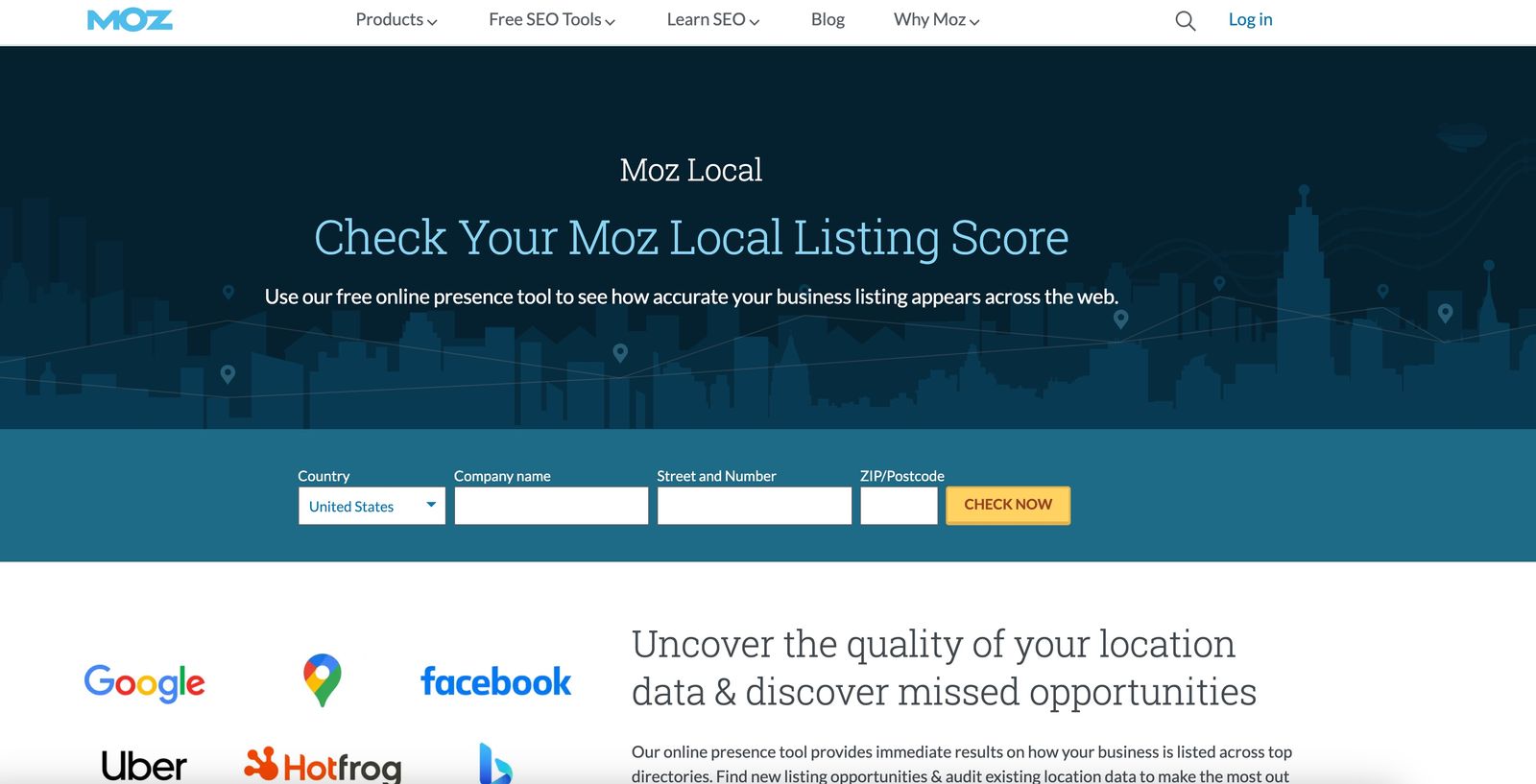This image is a screenshot from the website MOZ, prominently featuring a user interface designed to check a business's local listing score. At the top right corner, a login button is visible. The main content encourages users to "Check Your MOZ Local Listing Score" using their free online presence tool. This tool allows businesses to assess the accuracy of their listings across the web. 

There is a country drop-down menu with "United States" selected by default. Below this, fields are provided for entering company name, street address, and zip/postcode. The interface is adorned with logos from major platforms including Google, Facebook, Uber, Hot Frog, and Bing.

Adjacent to these logos, a text section invites users to "Uncover the quality of your location data and discover missed opportunities." The tool promises immediate results, helping businesses audit their current listings and find new opportunities across top directories. Unfortunately, the rest of the paragraph describing the benefits of the tool is cut off.